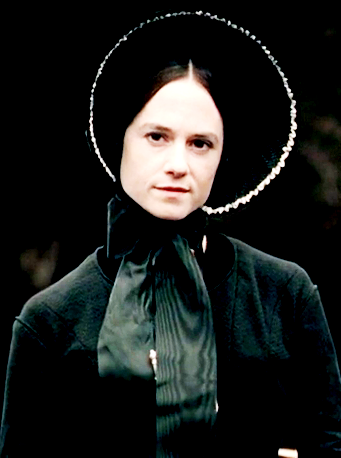This is a meticulously detailed photograph of a woman positioned centrally, making direct eye contact with the camera. She dons an elaborate black bonnet with a white trim and a substantial black bow tied beneath her chin, accentuating her square jawline. Her attire is completed with a dark, possibly Victorian-era jacket. The woman's hairstyle features a middle part, with her hair pulled back and concealed under the bonnet, which itself has a wide, circular brim framing her face.

The image, mostly rendered in monochromatic shades of black, white, and varying browns, exudes a historical or vintage aura, yet could plausibly be a modern-day interpretation of a 19th-century maiden, as seen in films like "The Piano." The woman's pale complexion is devoid of makeup, contributing to her austere and stern appearance, and she maintains a serious expression throughout. The background remains indistinct, reinforcing the focus on her figure. This professionally taken photograph leaves a strong impression of an old-timey, severe portrait, reminiscent of both pioneer and Victorian styles.